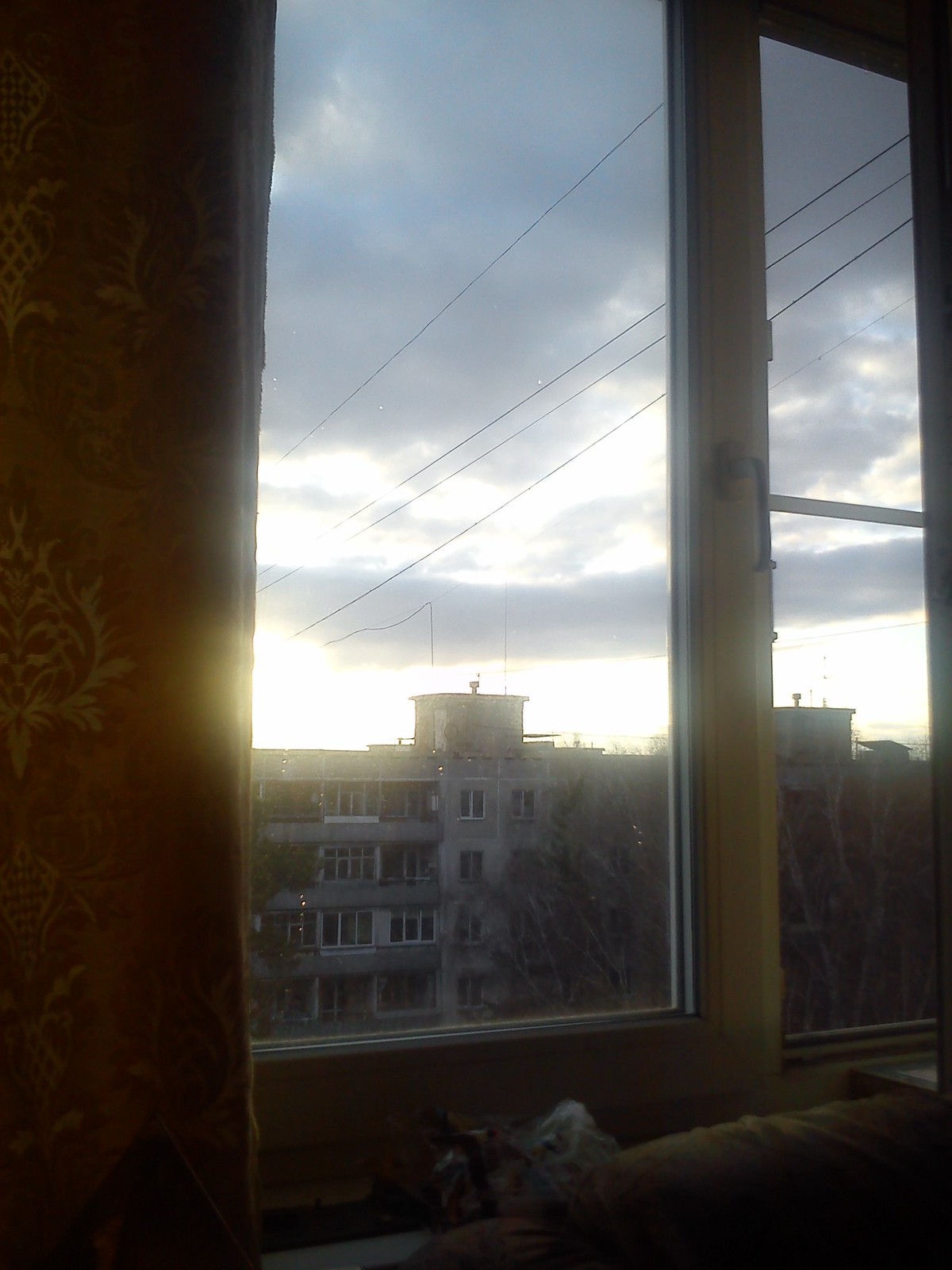The photograph captures an indoor view from an apartment, looking out through a set of glass windows with wooden frames and handles on the left side. Perched indistinctly on the windowsill at the bottom of the frame is an object that could possibly be a cat. The scene outside the window is set either during sunrise or sunset, giving the sky a grayish tone with interspersed dark clouds hinting at a potential storm. The horizon showcases a distant four-story white apartment building, complete with balconies on its first three floors, and is complemented by a few trees in the vicinity. To the right, partially visible through another smaller window with matching wooden frames, lies a neighboring structure. The foreground features power lines stretching diagonally across the view and a subtle paisley-patterned wallpaper on the interior wall to the left.